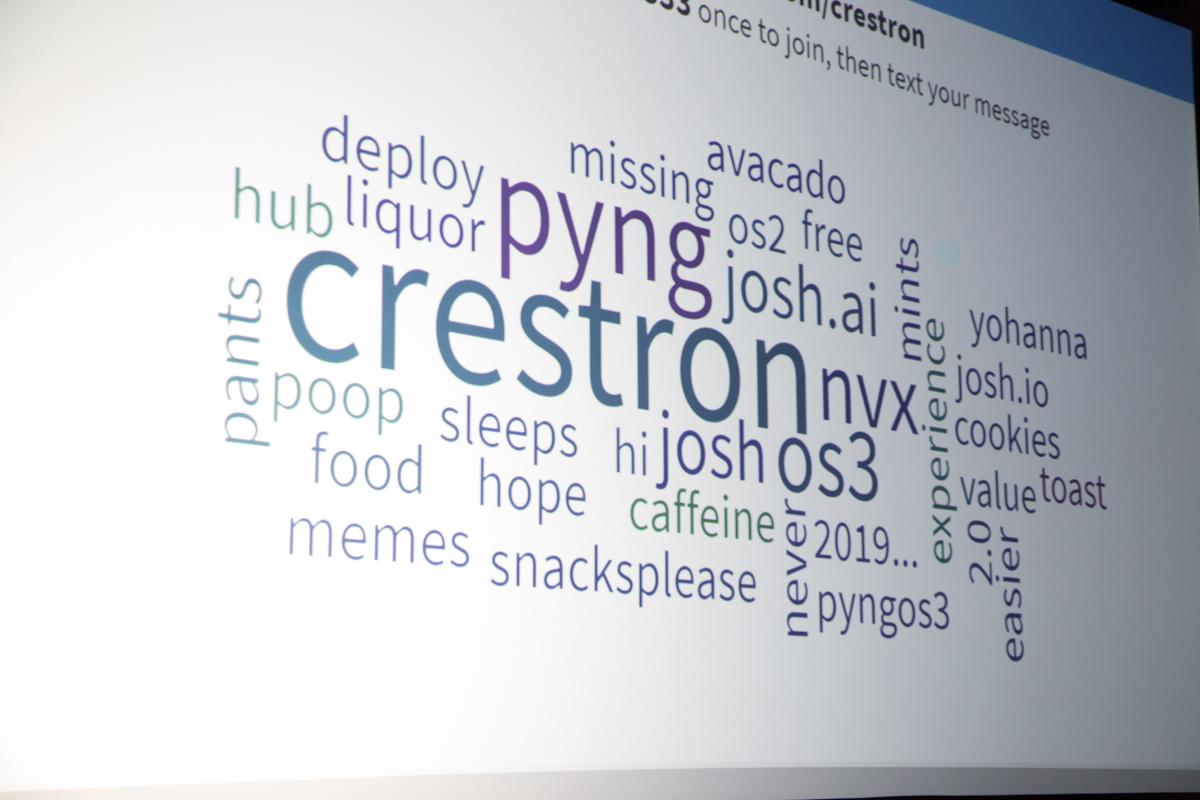The image depicts a presentation screen with a white background, displaying an intricate collage of words in various colors such as black, blue, teal, and green. Dominating the center is the word "Crestron" in large blue-gray lettering. Above it, "PYNG" appears in a purplish hue. Scattered around in different orientations—both horizontal and vertical—are a multitude of terms including "avocado," "missing," "deploy," "liquor," "hub," "poop," "food," "memes," "snacks please," "caffeine," "2019," and "Josh." To the right, there are words mentioning "cookies," "value toast," and "2.0." Additionally, words like "easier," "never," "experience," "mints," and "pants" are arranged vertically. At the top center of the screen, the lowercase letter sequence "C-R-E-S-T-R-O-N" is visible with light gray text underneath instructing "once to join then text your message." The overall arrangement creates a dense and colorful mishmash of assorted words and phrases.